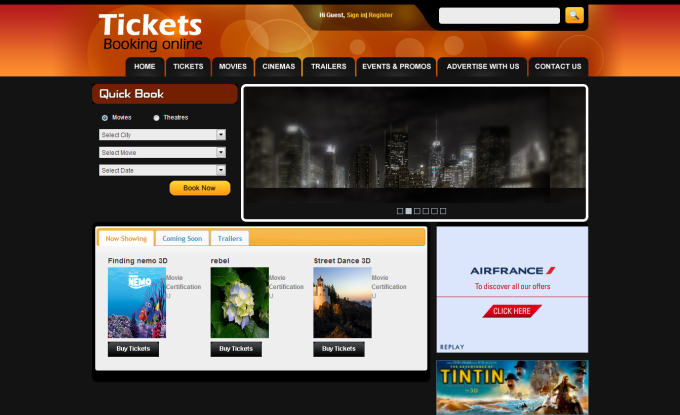This rectangular image, with its longer side extending horizontally, depicts an online ticket booking interface. At the top, there's an orangish-copper border displaying text that reads "Tickets, Booking Online" towards the left. Directly below this border, a row of tabs spans across the top of the interface, labeled uniformly in black with white text: "Home," "Tickets," "Movies," "Cinemas," "Trailers," "Events and Promos," "Advertise with Us," and "Contact Us."

To the top-right corner, the interface welcomes users with "Hi Guests," followed by options to "Sign In or Register." Adjacent to this, there is a white search box accompanied by a search icon.

Beneath this navigation area, there is a "Quick Book" link, followed by several fields allowing users to search for a city, movie, or date. Completing this section is a prominent yellow button with black text that reads "Book Now."

To the right of the search fields, there is a somewhat blurry image of a cityscape. Below this city image, there are advertisements for "Air France" and another ad seemingly related to "Tin Tin."